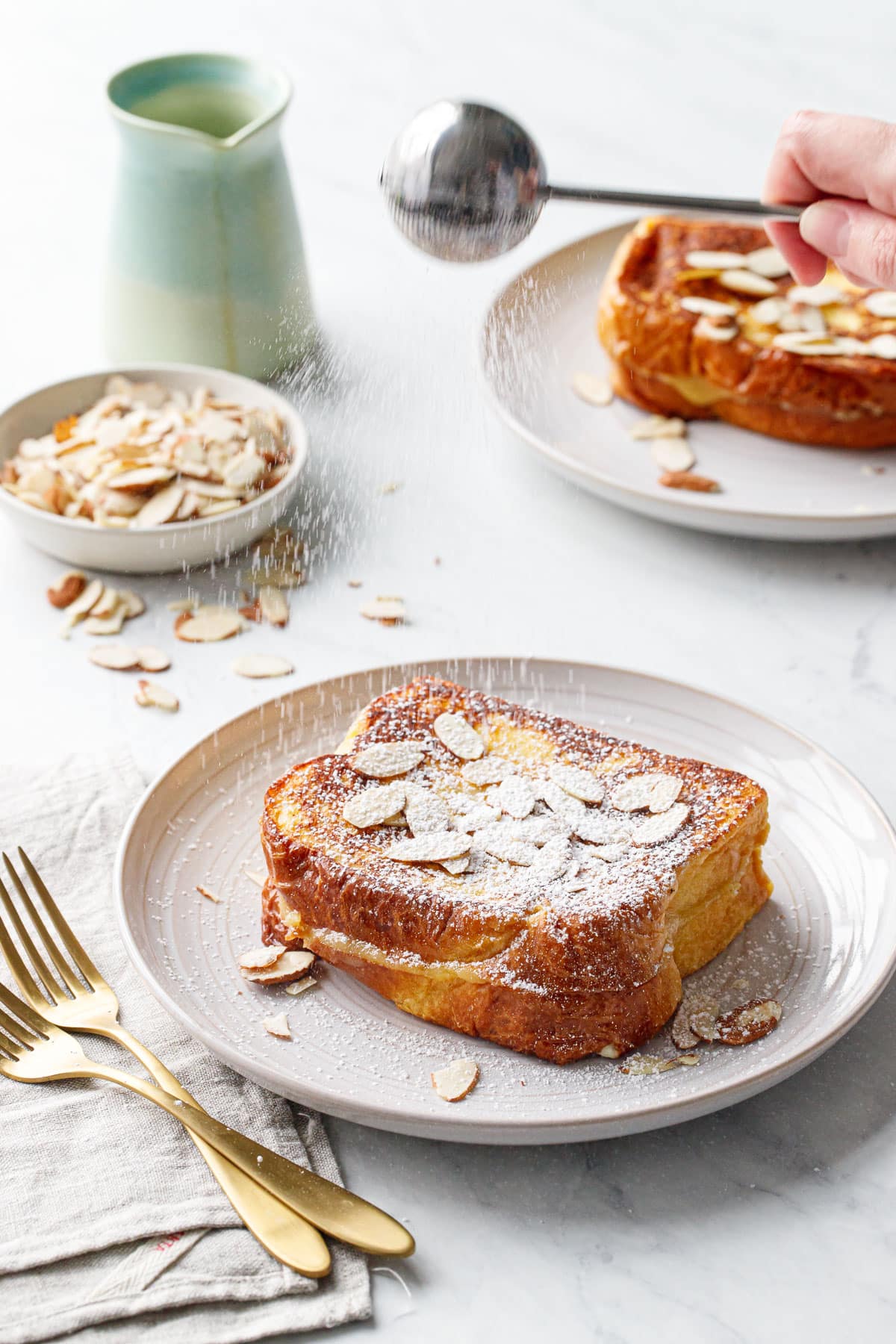The color photograph, likely taken for a recipe or cooking blog, features a portrait-oriented image centered on a white ceramic plate with a stack of two pieces of French toast. The French toast, adorned with sliced almonds, is being drizzled with powdered sugar from a silver sifter held by a woman's hand entering from the top right of the frame. The powdered sugar rains down like snow onto the toast. The plate sits on a light Carrara marble tabletop with a pale linen napkin to the left, upon which lie two matte or satin gold forks arranged neatly. In the upper left background, there's a low white bowl filled with sliced almonds, some of which have scattered around the table, and a blue and white clay pitcher with maple syrup visibly dribbling down its spout. Another plate of French toast with sliced almonds, awaiting its dusting of powdered sugar, is positioned in the upper right background.